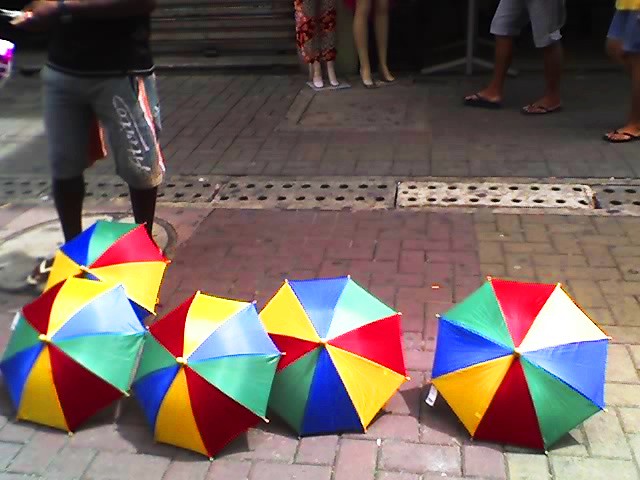In this vibrant outdoor street scene, five small child-sized umbrellas lie open and face the camera on a brick-paved sidewalk, resembling colorful beach balls with alternating triangles of red, yellow, blue, green, and white. The brick pavement, arranged in a basket weave or herringbone pattern, also features a manhole cover with a man standing on it. The man, visible from the mid-torso down, wears gray knee-length shorts, black socks with white flip-flops, and a black shirt. In the background, several passersby are visible, some wearing black flip-flops and others in different attire, like a woman in a long dress or skirt. Additionally, the legs of some mannequins can be seen standing outside a shop doorway, adding to the bustling, summertime atmosphere of the street.